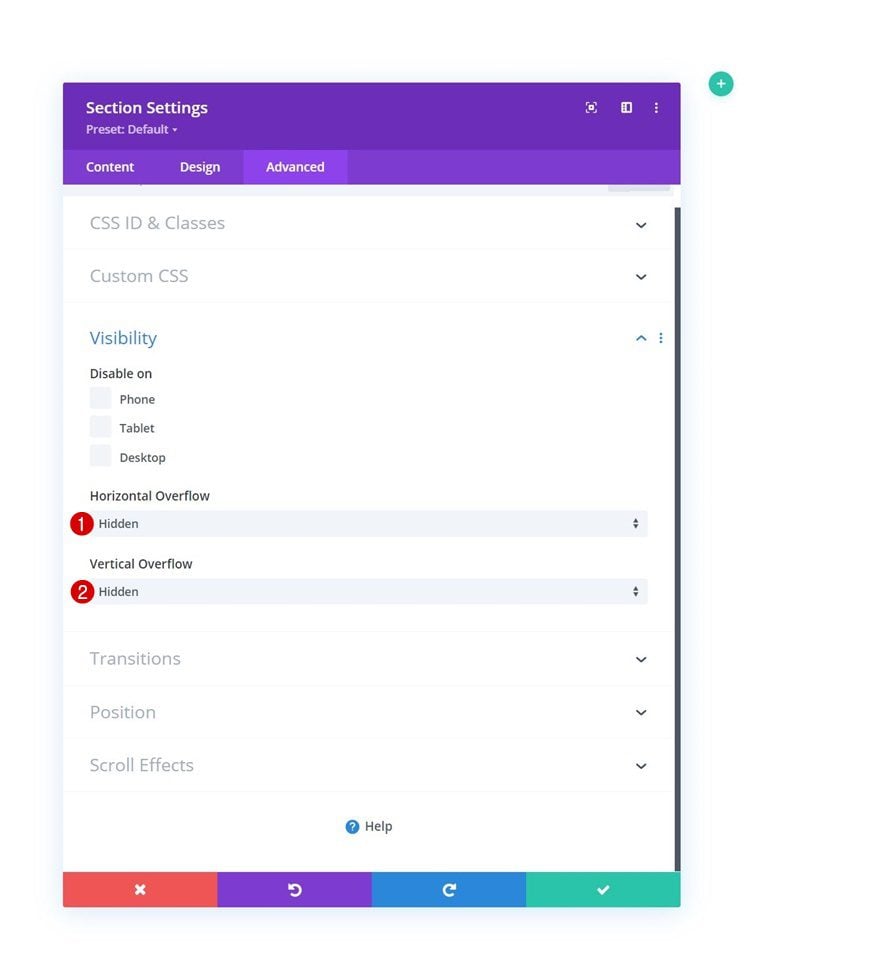The image depicts a "Section Settings" window with a sophisticated user interface design. The upper portion of the box is distinguished by a rich purple color, almost dark purple. The text "Section Settings" is prominently displayed in white font at the upper left-hand corner. Directly below this title, in a smaller white font, it reads "Preset: Default_".

Moving down, there is a lighter purple bar featuring a horizontal menu with three items in white font: "Content," "Design," and "Advanced." The "Content" tab is visually highlighted with a lighter purple square indicating it is the selected tab.

The main body of the settings box is white, featuring gray font for the various input fields and labels. The first section includes fields for "CSS ID" and "CSS Classes." Below this, there is a section labeled "Custom CSS."

Further down, the "Visibility" section is displayed with a drop-down menu that is currently open, showing options to disable the section on specific devices. Three checkboxes are present for "Phone," "Tablet," and "Desktop."

At the bottom, there is a section titled "Horizontal Overflow," detailing additional advanced settings.